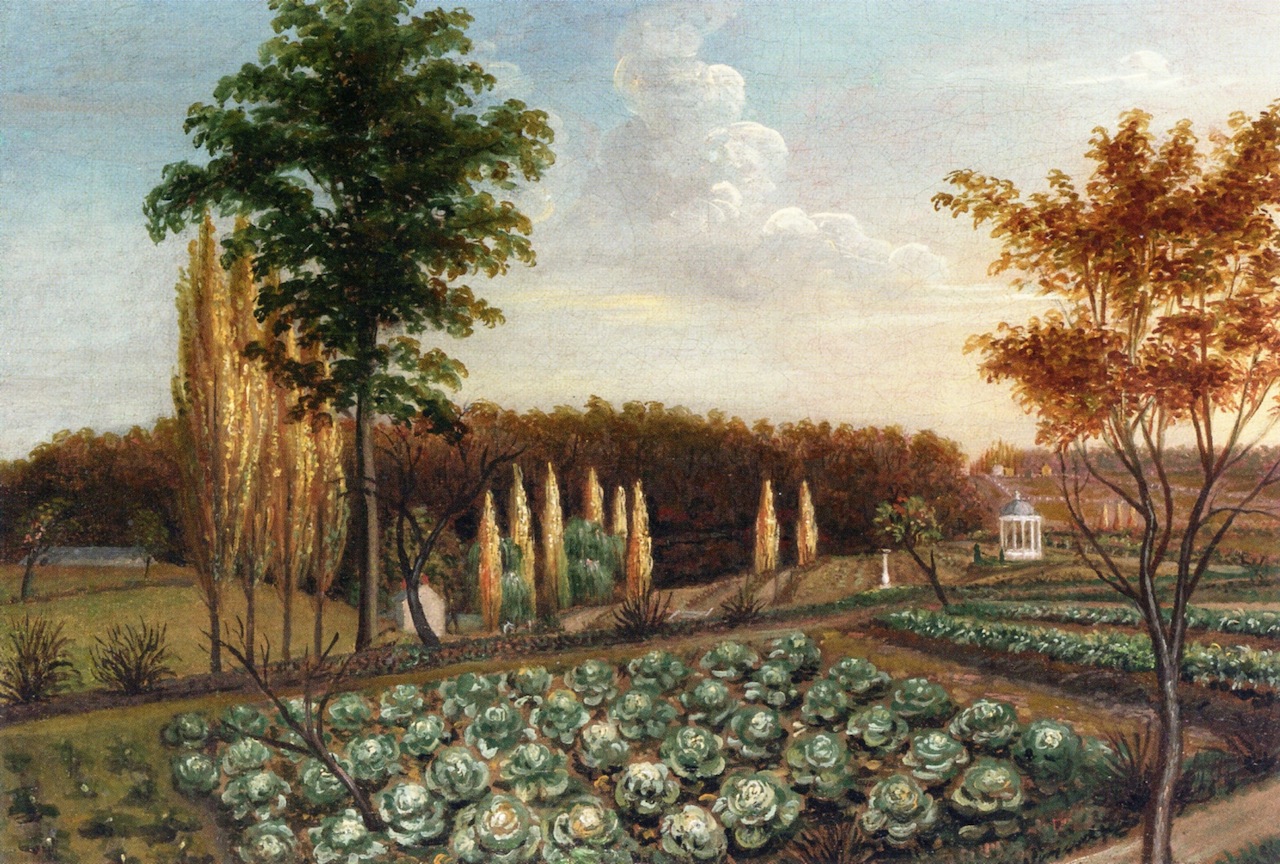The painting showcases a picturesque and well-manicured countryside garden scene. The foreground is dominated by rows of cabbages, thriving in the verdant field. Adjacent to the cabbages is a small, empty plot featuring green plants with brown leaves. Alongside this field, there winds a quaint dirt path that meanders through the landscape.

On the right side of the composition stands a tree with a thin trunk and slender branches adorned with yellow-orange leaves. Just to the left of this vibrant tree, a tall tree with a brown trunk and lush green foliage rises prominently. Interspersed among the greenery are several golden-leaved trees, some of which are tall and pointed, resembling evergreens bathed in autumn hues.

In the middle distance, a small stump rests near the cabbage patch, adding to the rustic charm. Behind the tall brown-trunked tree, there's a notable feature: a white building with a red roof, behind which sprouts another smaller tree with green foliage. Further back, more trees, including a grove with both golden and green leaves, compose a rich forested backdrop.

Towards the right of the scenery, amidst the lush vegetation, the elegant structure of a white gazebo with a gray domed top can be seen. This gazebo is flanked by pathways, one running perpendicular to the other, which hint at the careful planning of this idyllic garden layout.

The sky, painted bright and sunny, is dotted with puffy clouds, adding to the serene and inviting atmosphere of this tranquil countryside garden. Small homes or buildings are scattered in the distance, contributing to the overall peacefulness and charm of this landscape.